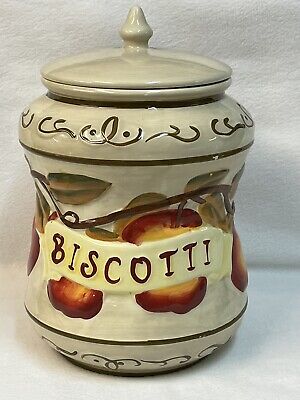This image features a ceramic cookie jar, centrally positioned and almost filling the whole frame from top to bottom. The jar is set against a white cloth backdrop, with subtle shading and wrinkles visible. The jar has a cylindrical shape with a slight wasp waist, tapering towards the middle before broadening out again. It has an off-white, cream-colored glaze and is adorned with intricate details.

At the top, the jar has a gray lid that resembles a mushroom cap, complete with a pointed tip and a noticeable black slit where the lid separates from the jar. Just beneath the lid, there's a gray rim featuring black squiggly designs reminiscent of plant stems. Below this, a slender gray line encircles the jar.

The center of the jar prominently displays a decorative branch bearing about five or six green leaves, along with two large apples rendered in red and yellow. A white banner with the word "biscotti" in elegant script crosses the middle of the jar, partially overlaying the apples.

Towards the base, a thin black line separates the central design from the jar's bottom section, which mirrors the top with its white base and black squiggly plant stem motifs. The overall artistic elements and detailed decorations give the jar a charming, rustic appeal.